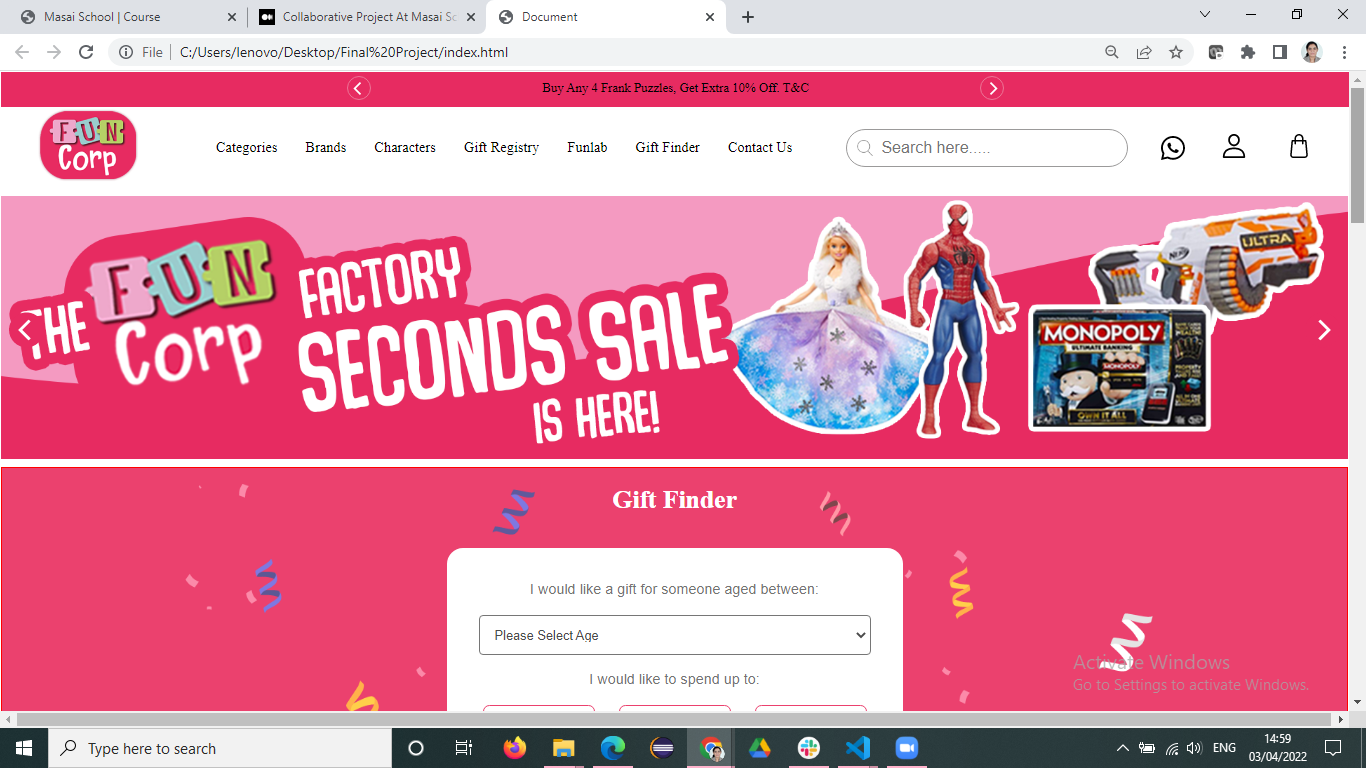An open web browser window on a computer running Windows 10 displays a project for a web design class. The screen features three open tabs, with focus on a tab labeled "document." The file path in the location bar reads "C: users/Lenovo/desktop/final project/index.html," indicating it's a local HTML file for a project.

The website, designed for a fictional company called FunCorp, prominently features a vibrant Barbie pink theme. FunCorp’s logo, creatively embedded into stylized jigsaw puzzle pieces with each letter in different colors (F in pink, U in turquoise, and N in green), is displayed at the top within a white band. This band also contains navigation links to various sections of the website, including Categories, Brands, Characters, Gift Registry, Fun Lab, Gift Finder, and Contact Us.

The main content area showcases a vivid Barbie pink announcement for Fun Factory Corp's "seconds sale," featuring a visually appealing layout. Key visual elements include images of a Barbie doll wearing a tiara and a blue starry dress, a Spider-Man figure, a Nerf machine gun, and a Monopoly game, emphasizing the fun and diverse products available.

Below this, a white pop-up interface within the pink section labeled "Gift Finder" invites users to specify details for a gift search. It includes dropdown menus for selecting an age range and buttons for setting a spending limit, although parts of these buttons are clipped out of view, suggesting typical gift amounts.

Overall, the project effectively showcases the student's web design skills, blending colorful and playful aesthetics with functional user interactions.